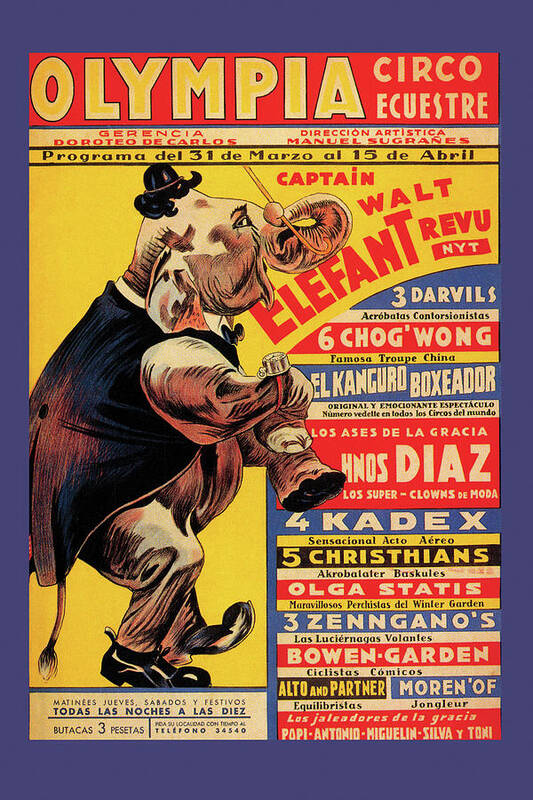This detailed poster, in portrait view, showcases an advertisement for the Olympia Circo Equestria event. Featuring a distinctive dark blue border and a striking red background, the title "Olympia Circo Equestria" is prominently displayed in bold yellow font at the top. Below the title, additional information about the event, including the program dates "Programma del 31 del Marzo," indicates that the circus runs from March 31st to April 15th.

Central to the poster's design is a whimsical illustration of an elephant. This elephant, poised on its hind legs, is adorned in an elaborate costume: a tiny top hat sits between its ears, complemented by a black wig. Its trunk deftly holds a cane. The elephant sports a black tuxedo with a long cloak, a white collar, and shiny black dress shoes, giving it a sophisticated appearance. The entire flyer is a vibrant blend of blue, yellow, red, and black, featuring an array of shapes and white text for additional details on the right-hand side. The artistic and colorful composition effectively captures the circus's lively and magical atmosphere.